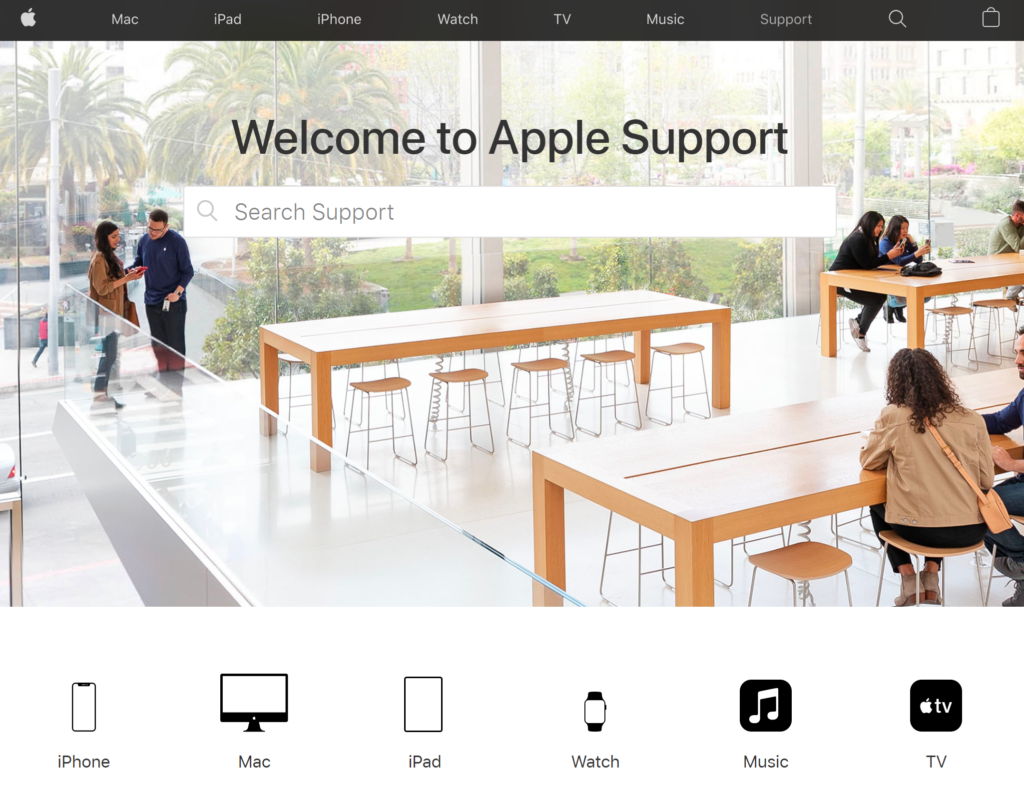The image features an Apple Support page with a prominent, large black text in the center that reads, "Welcome to Apple Support." The photo is an overlay, with the background displaying lush greenery including palm trees, grass, and shrubbery, reminiscent of a garden or yard. Inside the foreground, there are three long wooden tables, each flanked by five stools on either side. The wood of the tables is light in color, giving off a modern aesthetic.

At the first table, all the stools are neatly pushed in, and no one is seated. However, nearby stand a man and a woman. The man, sporting dark hair, glasses, and dressed in dark attire, is engaged in a conversation. The woman, with dark hair, wearing a tan blazer and black pants, faces the table and appears to be showing something on her phone to the man, whose back is to the table.

Moving to the far right table, two women are seated together, alongside a partial view of a man's shoulder, indicating his presence. Lastly, at the nearest table, a man and a woman are seated opposite each other. The scene is framed by the welcoming message of Apple Support, inviting users to the friendly and engaging environment of the support area.